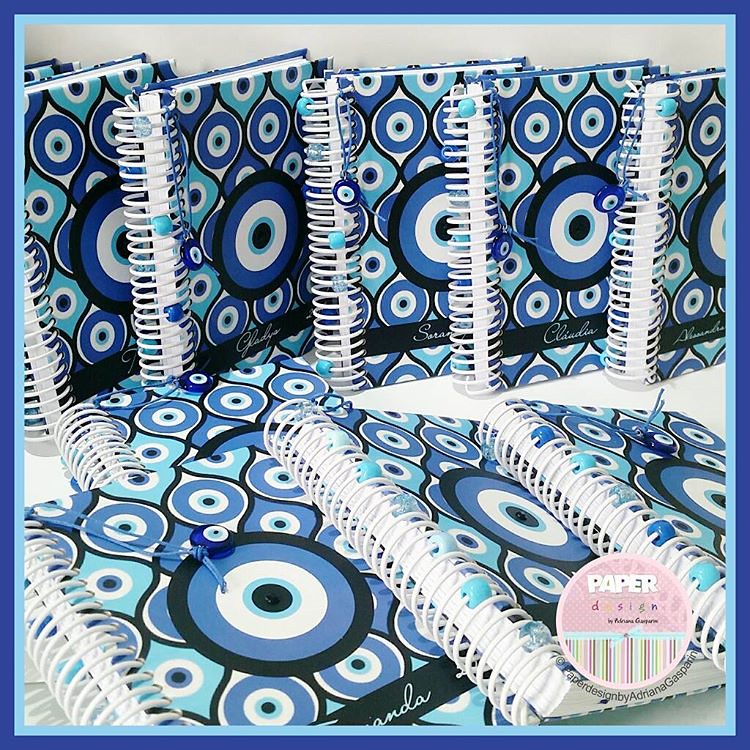The image depicts nine spiral notebooks, all with identical covers and features. The notebooks are arranged with four on the ground and five standing vertically. Each notebook sports a white spiral binding on the left side and a cover adorned with a series of concentric circles, predominantly in shades of blue—ranging from baby blue to dark blue—and black. At the center of each cover is a large, stylized black circle encircled by successive rings of baby blue, white, and medium blue. Scattered across the blue and white cover background are smaller circles mirroring the central design. Adding to the design, a small logo in the bottom right-hand corner features the word "paper" in white text against a two-tone backdrop of pink and multicolored thin lines. The notebooks are likely set on a white table, evidenced by the visible white surface, with a gray-tinted background at the top of the image.